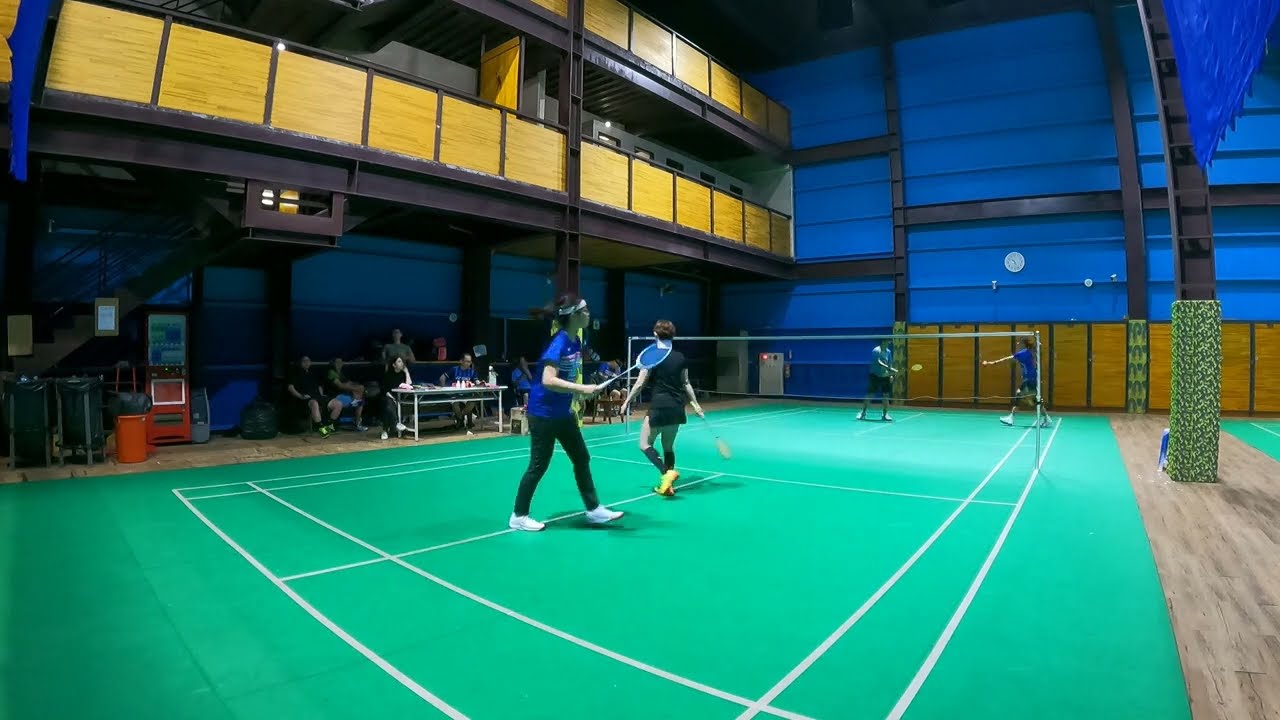The image depicts an indoor badminton court inside an aluminum building structure characterized by its blue walls and various color details. The bright green court, divided by white markings, is the focus of the scene. A match is underway with two players on each side of the net, all wielding badminton rackets. The players' attire includes blue, black, and possibly light gray tops. To the left, a balcony or gallery area hosts spectators, some seated at tables and in chairs, giving the impression of an audience or participants in a competition or practice session. Above this area, there are multi-level hallways. Cushioned support posts, painted a vibrant yellow, are visible, indicating safety features. Additionally, large windows and bright lights are noted, suggesting it's nighttime. The surrounding area consists of green, blue, yellow, tan, and other colors, creating a vivid and lively indoor sports setting.